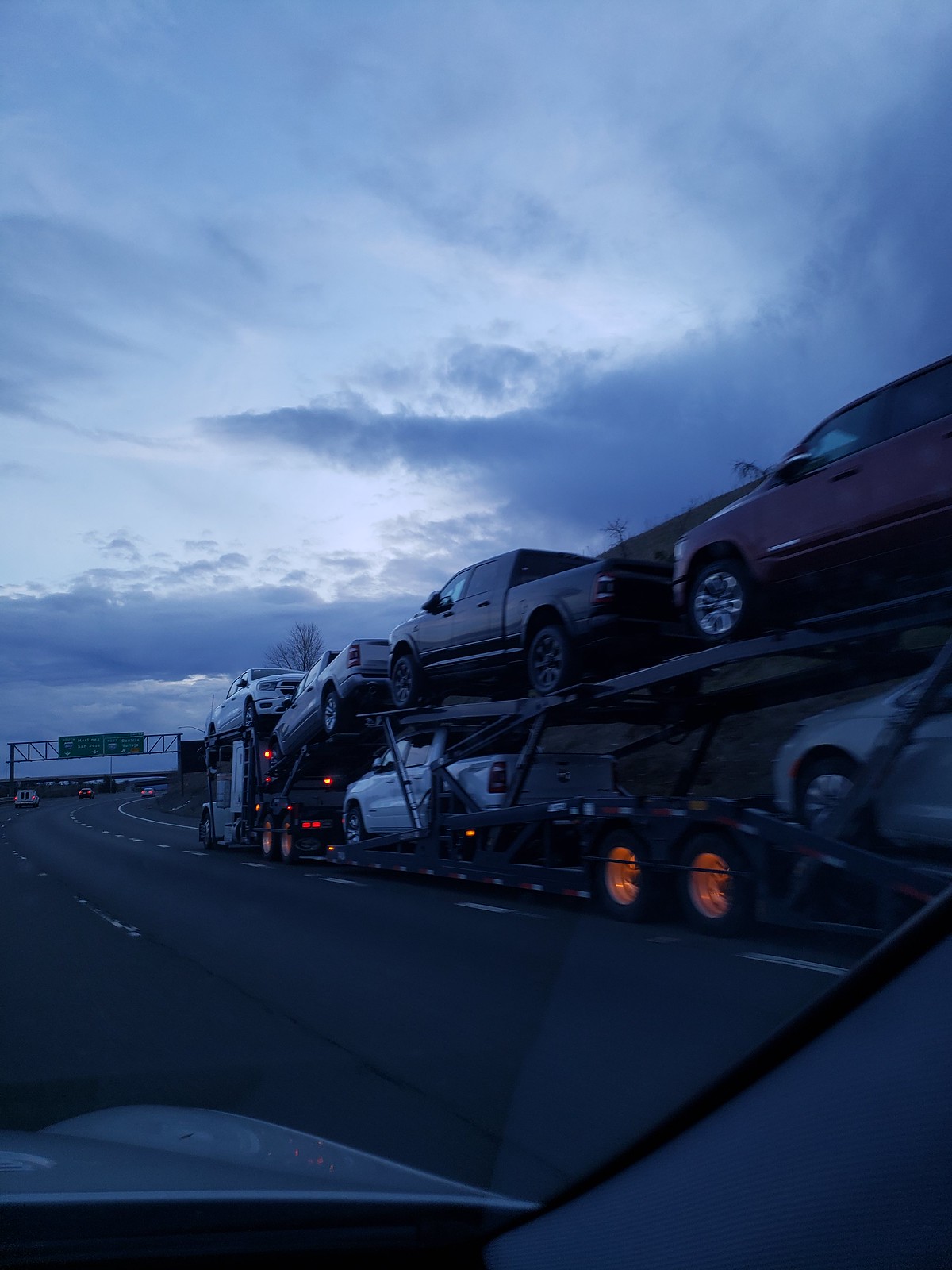The image depicts an evening scene taken from the front window of a car traveling down a highway. The sky is dark with large, wispy clouds, indicating it is either dusk or heavily overcast. To the right of the car, two lanes over, is a white 18-wheel car carrier truck, its orange-lit wheels illuminating the road around it in a peculiar manner. The trailer is stacked with a total of seven pickup trucks: four on the top rack and three on the bottom. The trucks vary in color, including white, silver, deep red, and black. In the distance, a green road sign is visible, giving directions. The highway curves ahead, marked by white lines on the dark, tinted blue pavement, reinforcing the moody, dimly lit atmosphere of the scene.